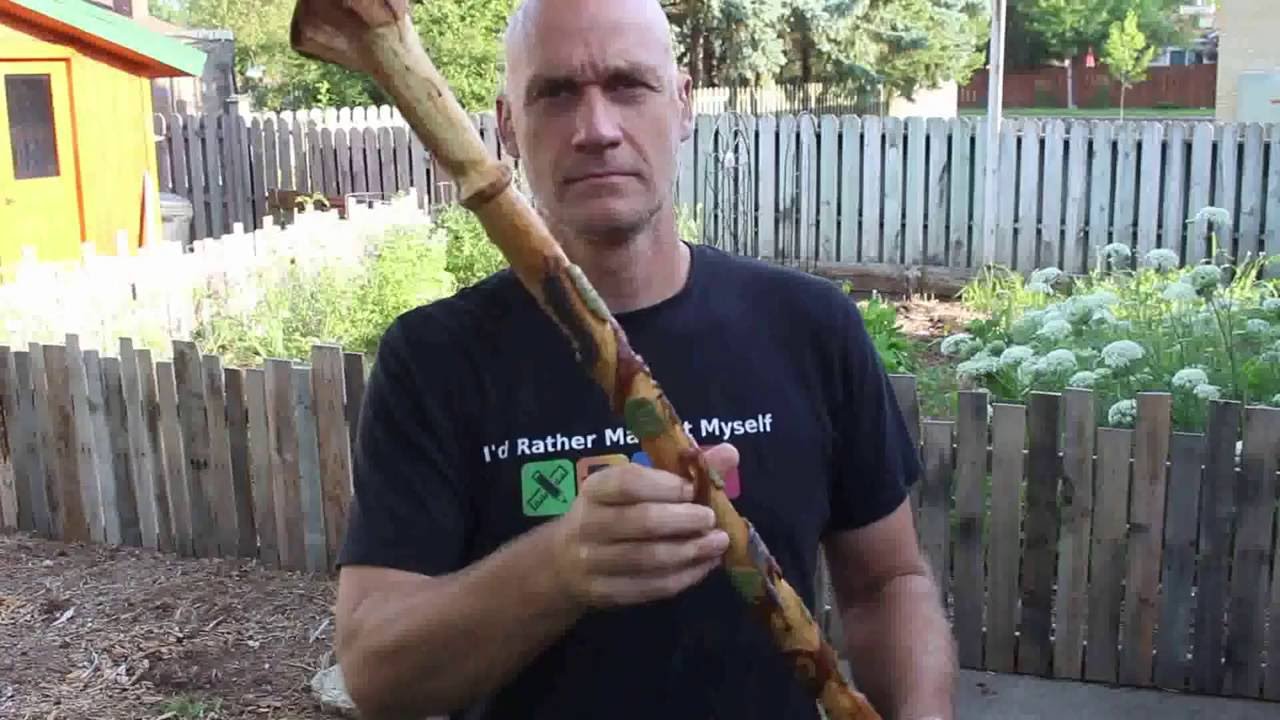The photograph displays a middle-aged Caucasian man, possibly in his early 40s to 60s, with a bald head and a fit physique, standing outdoors in a yard. He is wearing a navy blue t-shirt with a partially obscured white text that reads "I'd rather make it myself." The man appears to have a serious or slightly frustrated expression, possibly due to the sun's glare. He is holding a long wooden artifact that is intricately carved and decorated with colorful designs, predominantly green and burgundy. The setting is a fenced yard with visible grass, flowers, and plants, suggesting a garden environment. Behind him, there is a small yellow structure that could either be a shed or a house. The background includes additional fencing and what seems to be a neighborhood area beyond the yard.